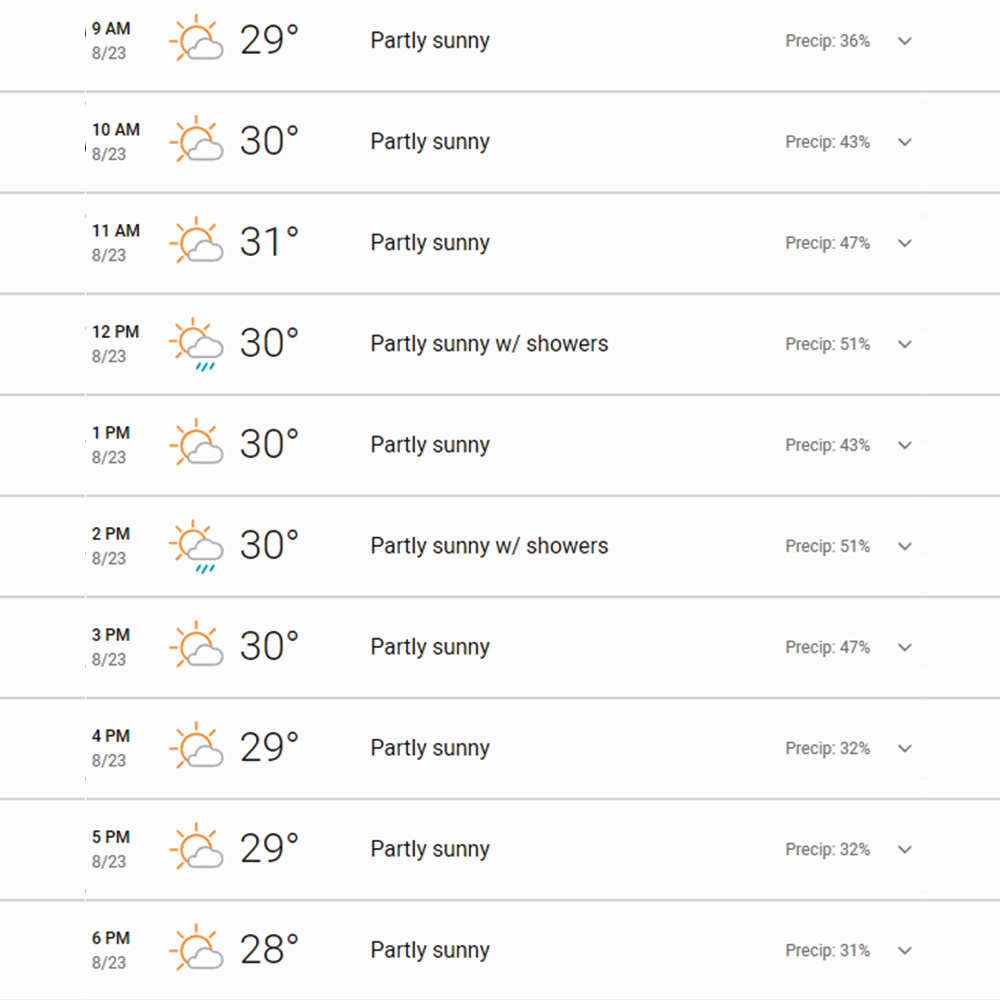A detailed weather forecast is displayed on a weather app interface. The forecast is organized in a column format, divided by lines representing each hour of the day from 9 a.m. to 6 p.m. 

- **9 a.m.:** The weather icon shows a sun partially obscured by a white cloud, indicating partly sunny conditions. The temperature is 29 degrees. The precipitation rate is 36%, with a downward-pointing arrow suggesting decreasing likelihood.

- **10 a.m.:** The icon remains the same with a sun and cloud for partly sunny skies. The temperature rises to 30 degrees. Precipitation probability climbs to 43%, still accompanied by a downward arrow.

- **11 a.m.:** Partly sunny conditions persist with the same icon, and the temperature remains at 30 degrees.

- **12 p.m.:** The weather changes slightly to partly sunny with showers, as depicted by a sun, cloud, and rain droplets. The temperature is 31 degrees.

- **1 p.m.:** It returns to partly sunny, with the temperature maintaining at 31 degrees.

- **2 p.m.:** Once again, it shows partly sunny with showers. The temperature remains steady at 31 degrees.

- **3 p.m. to 6 p.m.:** The forecast reverts to partly sunny for the remainder of the day, with the temperature hovering around 31 degrees and slight fluctuations in precipitation percentages.

This detailed hourly breakdown allows users to anticipate weather changes throughout the day, providing helpful information for planning activities.